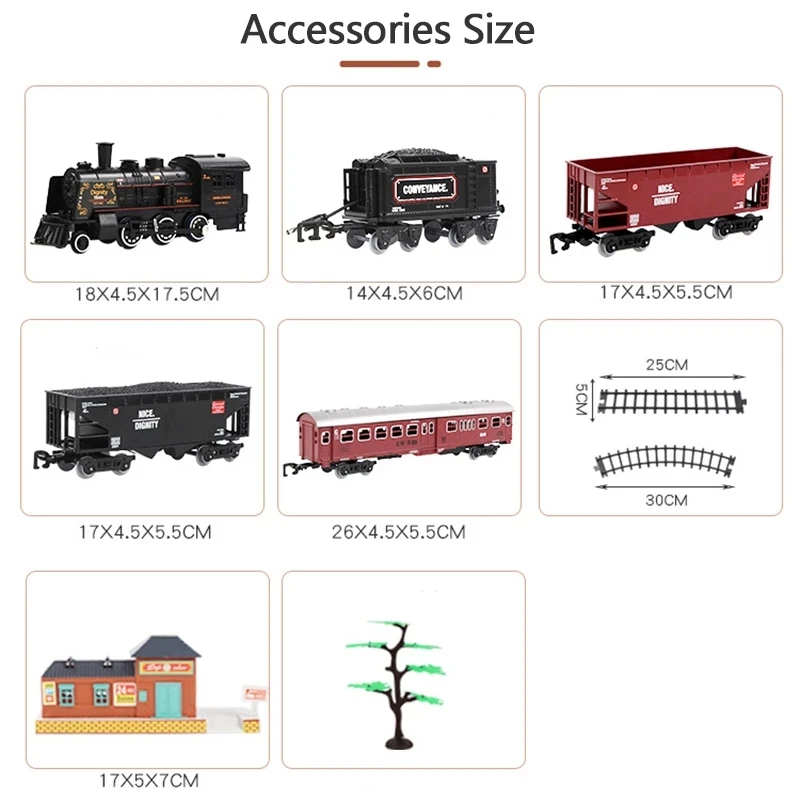This detailed image showcases a collector's toy train set, complete with accessories and dimensions. Clearly labeled at the top in black text, it reads "accessories size," followed by a thin brown line. The layout consists of eight squares—three at the top, three in the middle, and two at the bottom—each framed with a light brown border and housing a white background featuring a component of the train set alongside its dimensions. 

In the top left square, there's a toy locomotive measured at 18 by 4.5 by 17.5 centimeters. Adjacent to it, in the middle top square, is a toy coal car, 14 by 4.5 by 6 centimeters. The top right square displays a red train carriage, 17 by 4.5 by 5.5 centimeters. In the middle row, from left to right: the left square houses a black carriage of the same dimensions (17 by 4.5 by 5.5 centimeters), the center square features a red and white passenger carriage measuring 26 by 4.5 by 5.5 centimeters, and the right square displays two types of train tracks—straight tracks at 25 centimeters long and curved tracks at 30 centimeters. 

At the bottom, the left square shows a brick train station with a green door and black roof, measuring 17 by 5 by 7 centimeters. The final square, positioned in the middle bottom, contains a decorative tree with green leaves, though it lacks specific measurements. This thorough portrayal provides train collectors with precise details about each accessory included in the train set.